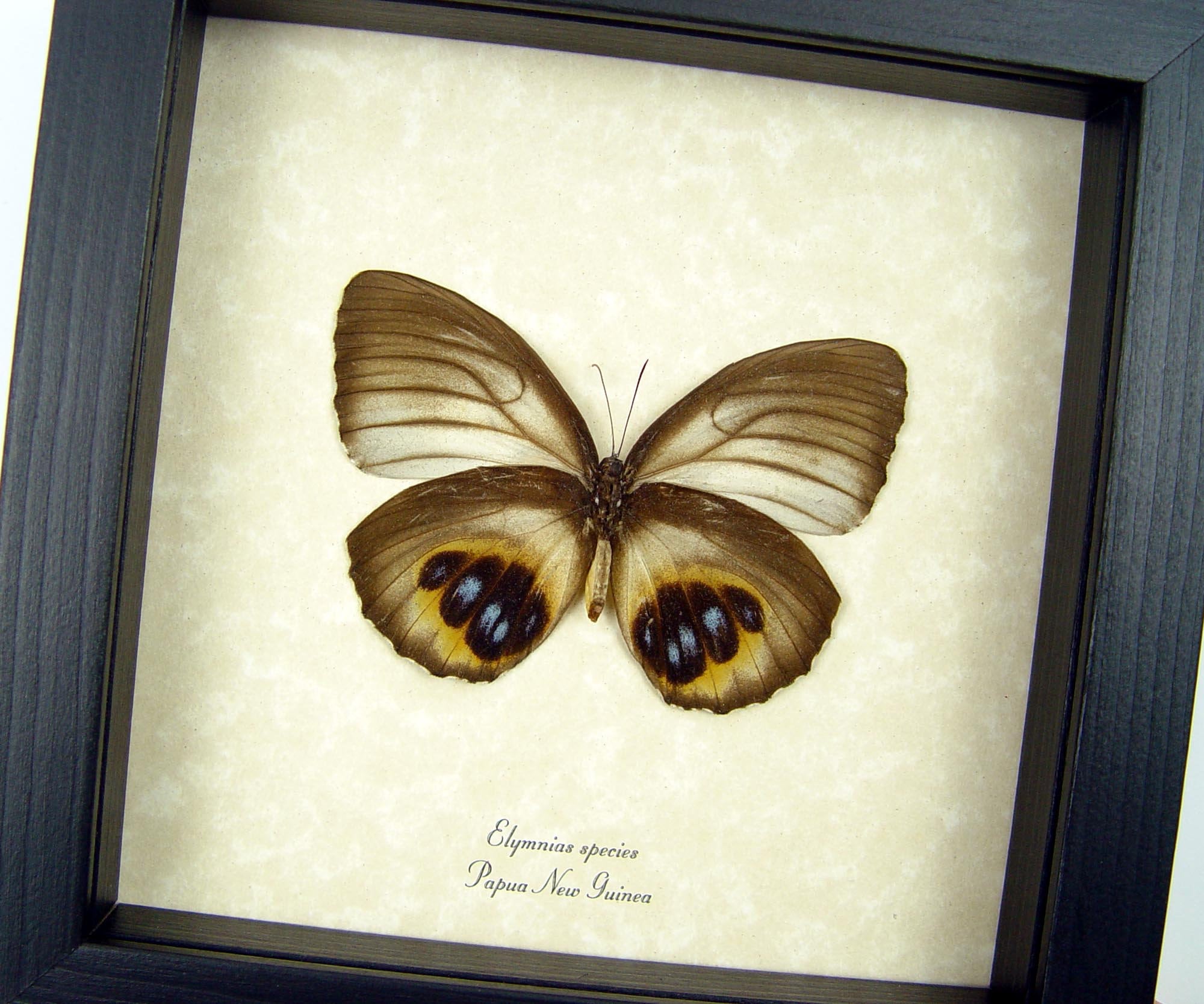The image depicts a framed exhibit of a detailed butterfly, or possibly a moth, labeled as "Illumina species Papua, New Guinea." The creature is displayed in the center of a piece of beige paper within a black, wooden, square frame. The butterfly's wings are spread wide, showcasing a predominantly brown color palette accented with beige, yellow, and black. Notably, the black sections of the wings feature small blue circles. The insect's anatomy is clear, with two long antennae, visible veins on the upper wings, and distinct lower wings adorned with blue splotches over yellow patches. The insect appears well-preserved and is covered with protective glass, emphasizing its exhibition style.